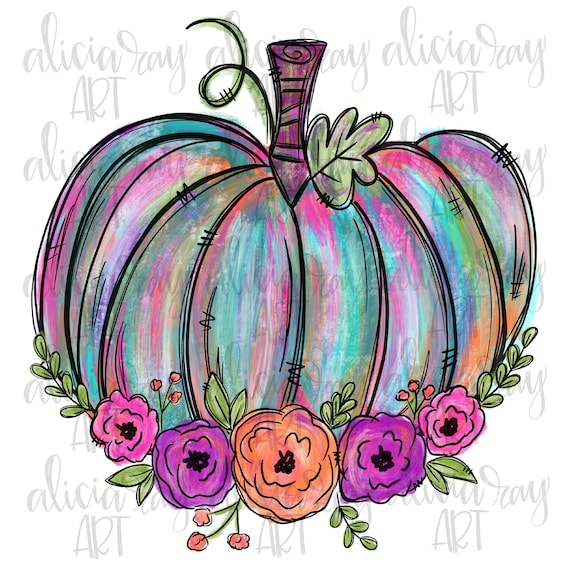"This vibrant watercolor artwork by Alicia Ray Art features a colorful pumpkin positioned centrally on a white backdrop with light gray watermarks of the artist's name. The pumpkin showcases a palette of evening shades, including purple, blue, green, yellow, and pink, and is outlined in black. It has a brown stem with a green leaf and a delicate green tendril sprouting from the top. At the base of the pumpkin, there is a beautiful arrangement of five peonies in pink, purple, and orange hues, surrounded by lush greenery. The detailed brush strokes vividly bring out the texture and richness of the colors, creating a visually striking piece."